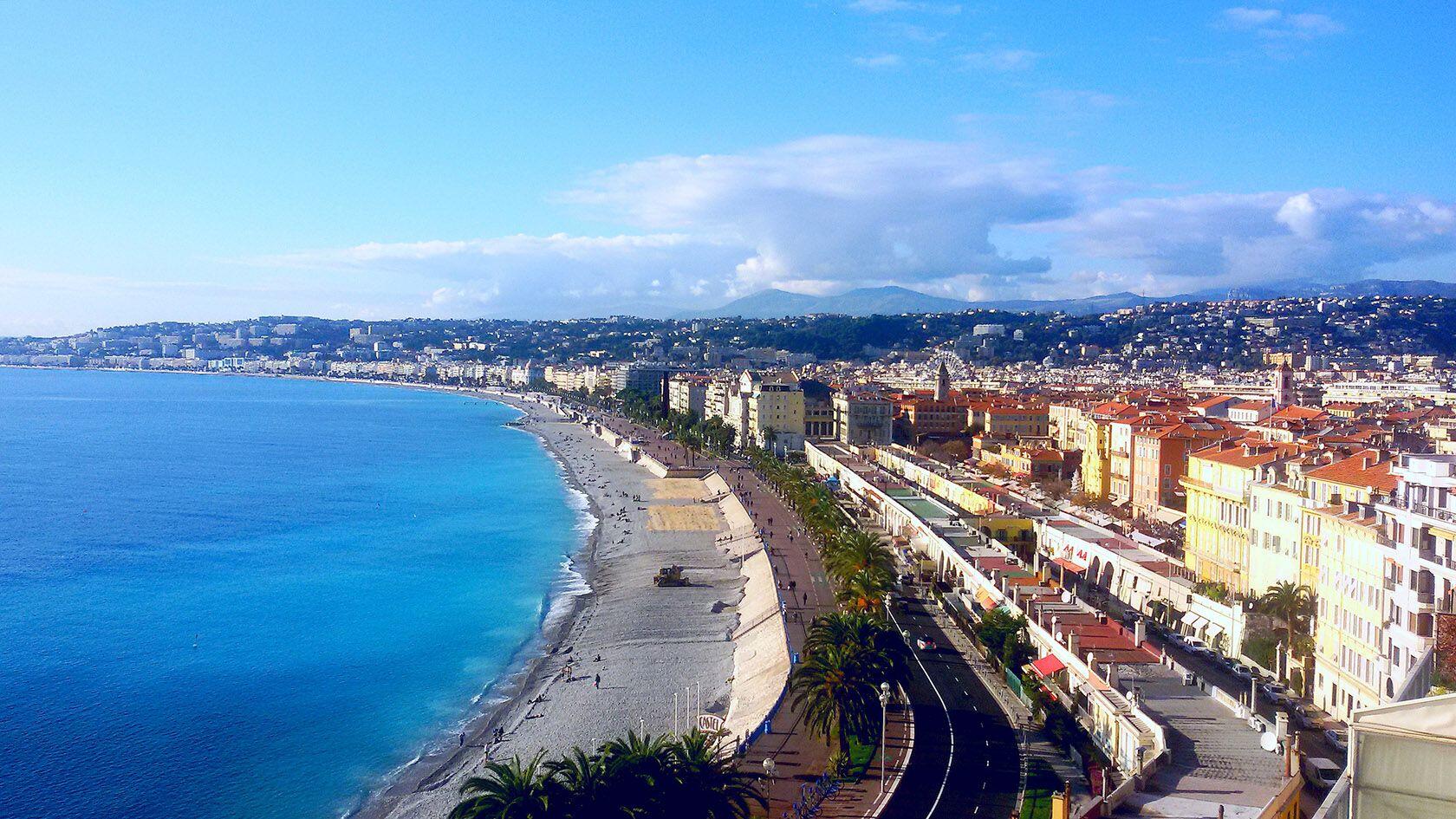A vibrant aerial photograph captures Nice, showcasing the iconic Promenade des Anglais along the stunning Mediterranean coast. On the left, the shimmering blue ocean merges into light gray sandy beaches sprinkled with beachgoers. The shoreline transitions into a bustling cityscape filled with palm trees and various architectural styles. A black asphalt road with white divider lines runs parallel to the beach, accompanied by a busy boardwalk. The right side is dominated by colorful apartment buildings adorned with yellow, salmon, and white façades, topped with red clay tile roofs. In the distance, a ferris wheel adds to the charm as it presides over the cityscape. The backdrop of majestic mountains is visible under a bright blue sky dotted with white clouds, completing this picturesque coastal scene.